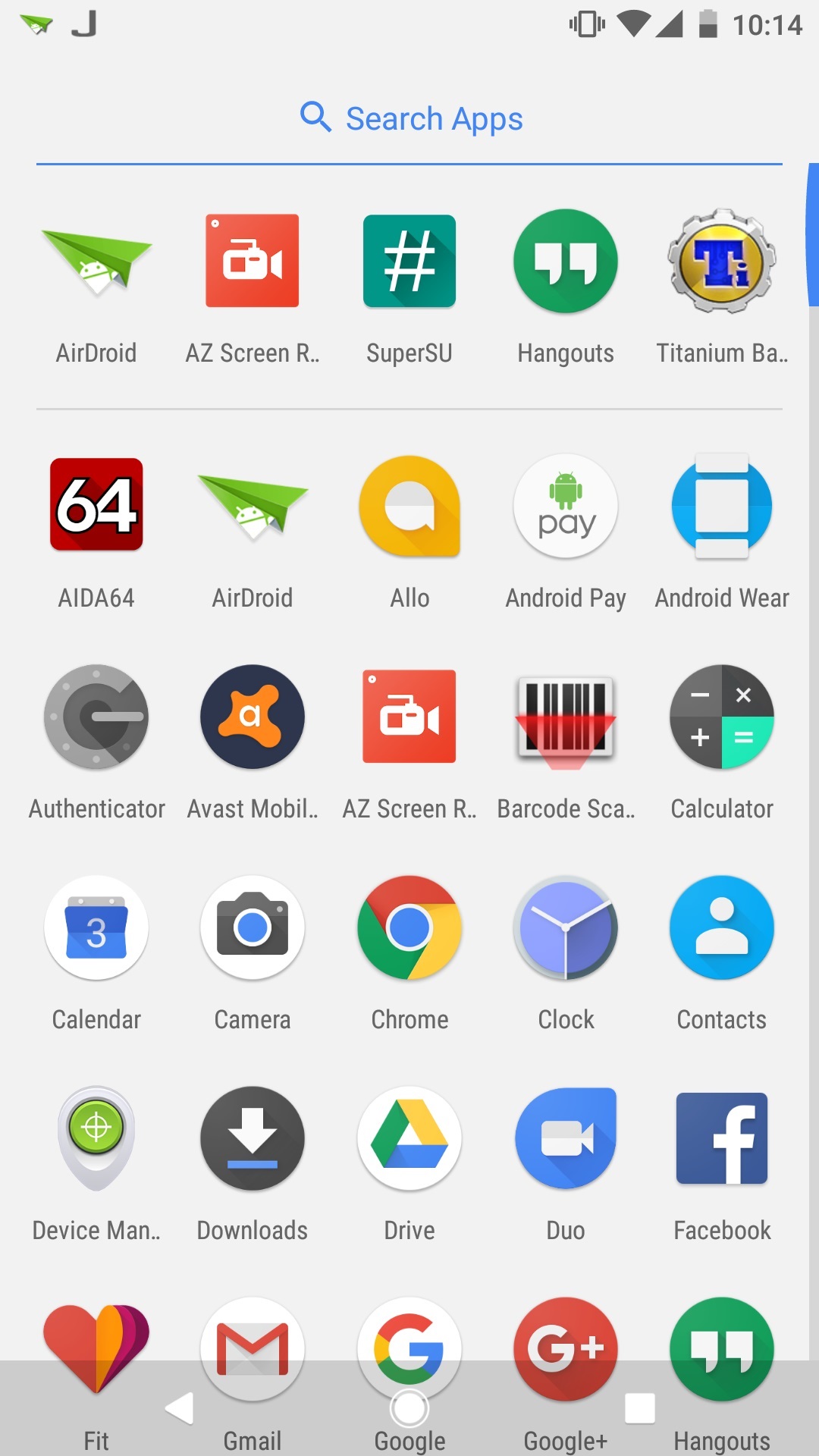This image is a screenshot from a smartphone, set against a very light gray background. In the upper right corner, the time reads "10:14," though it does not specify whether it is a.m. or p.m. The battery icon indicates it's about half charged. Additional icons show the status of the wireless connection, Wi-Fi connection, and that the phone is on mute.

At the top center, "Search apps" is written in blue font, accompanied by a blue circular search icon with a diagonal line extending downwards to the right. Below this, the screen displays a grid of various app icons, organized into five columns and six rows.  

The top row includes apps such as "Android," "AZ Screen Recorder," "SuperSU," "Hangouts," and "Titanium Backup," though some app names are truncated with ellipses. The icons are diverse and colorful, including a red square icon with bold white numbers "64," the Chrome logo, Google Drive logo, and Gmail logo. Notably, this screenshot includes some older or now-defunct apps like Google+, alongside other familiar apps such as Facebook, Hangouts, Contacts, Calendar, and Camera.

Overall, the screen showcases a wide variety of applications, reflecting a typical, albeit somewhat dated, organization of a user's app collection.